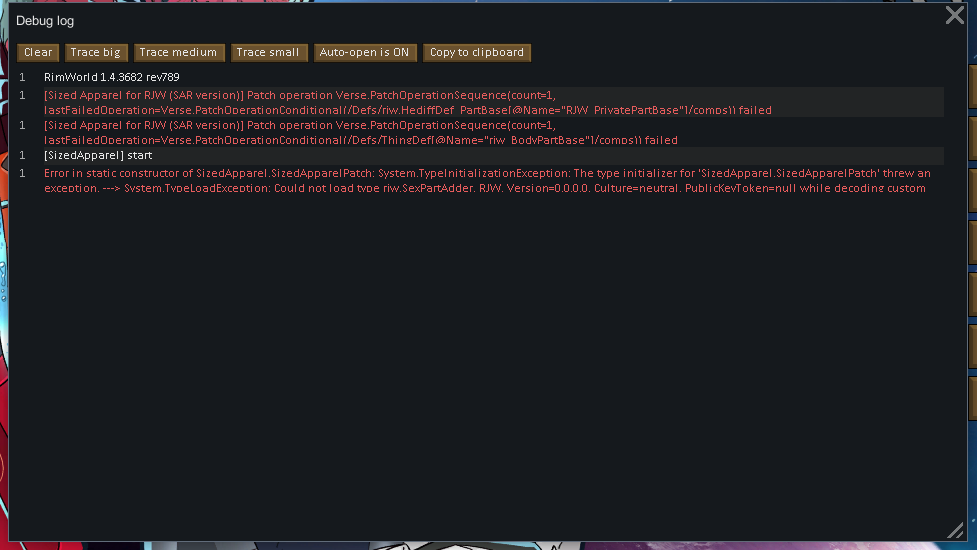This image is a screenshot focused on a debug log displayed prominently in the foreground, obscuring most of the underlying elements. The debug log occupies nearly the entire screen, save for a light gray 'X' in the top right corner that likely serves as a close button.

The background of the image gives off a colorful yet blurred impression, possibly depicting an anime-themed wallpaper on a laptop, with hues of blue, red, gray, and purple faintly visible. The debug log window itself is divided into several sections. At the top, enclosed in brown rectangles, are labeled options: Clear, Trace Big, Trace Medium, Trace Small, Auto-Open (highlighted in capital letters), and Copy to Clipboard.

Below this toolbar, a line of white text reads: "RimWorld 1.4 3682 REF 789." Following this line, the log lists various entries, each prefixed with the number "1" and then specific debug information enclosed in brackets and different colored text. Particularly notable is a red entry.

The error logs detail specific issues encountered within the program. One critical error reads: "Error in static constructor of SizedApparel, SizedApparelPath: System.TypeInitializationException: The type initializer for 'SizedApparel.SizedApparelPatch' threw an exception —> System.TypeLoadException: Cannot load type 'RimWorld.SexpArtAdder'," followed by additional error messages and technical specifics.

In summary, this detailed screenshot not only provides a glimpse into the specifics of a debug process for the game RimWorld but also hints at both the user's aesthetic desktop choices and the technical hiccups faced during development or modding processes.